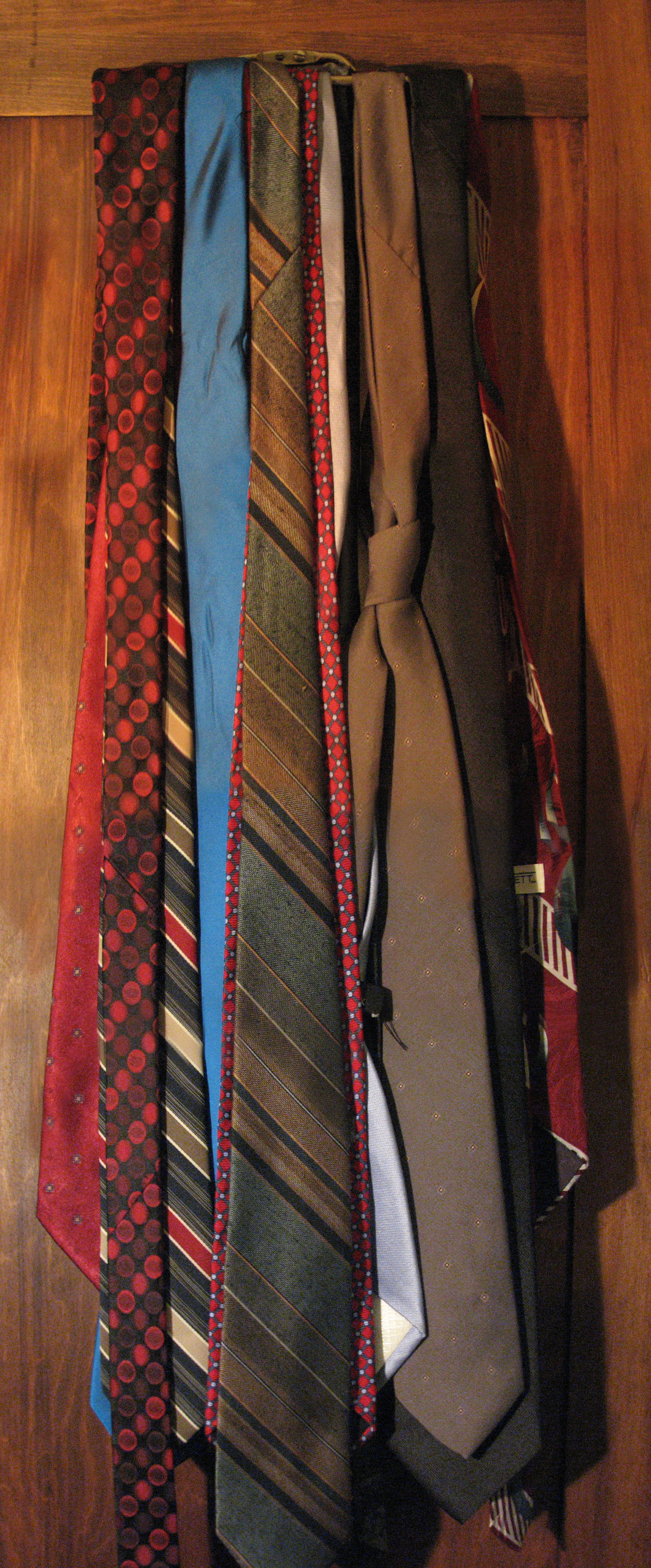The image is a vertically oriented rectangle featuring a collection of men's ties hanging from a ledge against a brown wooden wall. The ties, which are well-lit with a shadow cast to the right, exhibit various styles and colors. From left to right, there is a red tie with white dots, a black tie with red dots, a tie with stripes in gray, black, brown, white, and red, a solid blue tie, a tie with dark gray, dark brown, and light brown metallic stripes, a solid dark brown tie, a plain solid black tie, and another tie that is black with red patterns. The arrangement appears vintage, showcasing a diverse array of ties in typical patterns and solid colors.